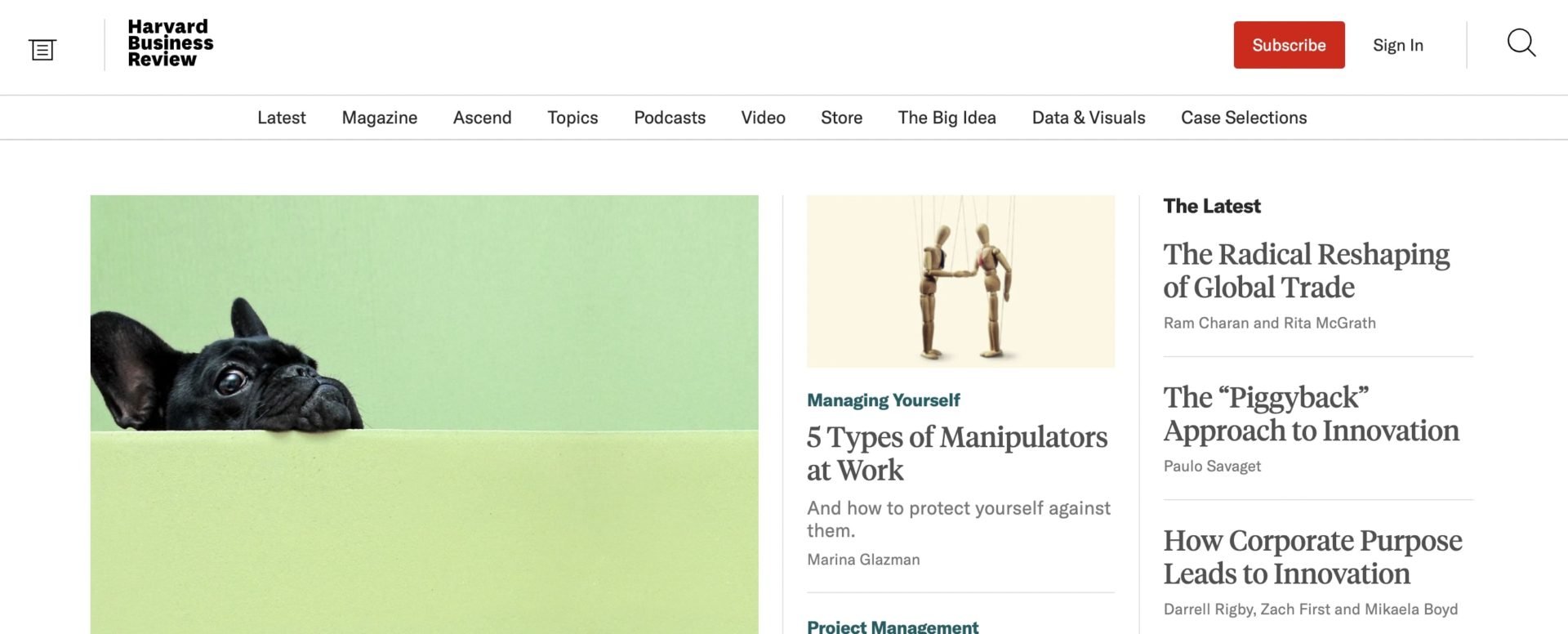The top left corner of the image features the text "Business Review" in black writing. To the right, there's a red rectangle labeled "Subscribe." Adjacent to that is the "Sign In" option, followed by a magnifying glass icon for the search bar in the top right corner. Below this header, a menu bar extends with ten categories arranged from left to right: "Latest," "Magazine," "Ascend," "Topics," "Podcasts," "Video," "Store," "The Big Idea," "Data and Visuals," and "Case Selections."

In the bottom left corner of the image, there is a small black dog's face peeking out from under an object, gazing upward towards the top right. The background directly beneath this image is a vibrant lime green, transitioning to a leafy green color above it.

To the right of the dog's image, there is an article titled "Five Types of Manipulators at Work," accompanied by a picture featuring a light pink background with two brown action figure statues. Further to the right, a section labeled "The Latest" lists three articles with a white background. The top article is "The Radical Reshaping of Global Trade," followed by "The Piggyback Approach to Innovation," and the third, "How Corporate Purpose Leads to Innovation."